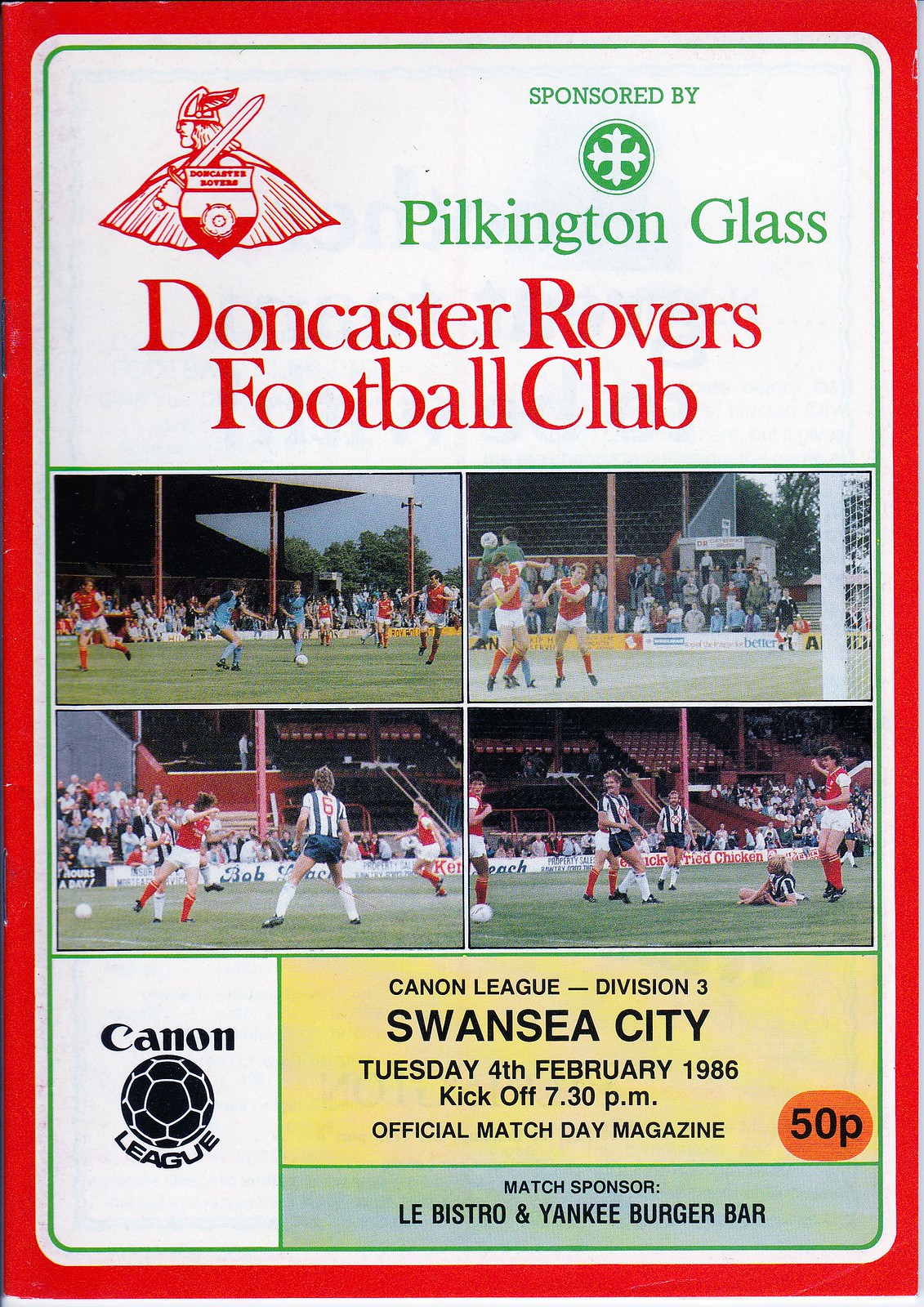This detailed advertisement for a soccer match features a bold red border enclosing the entire ad, which is sponsored by Pilkington Glass for the Doncaster Rovers Football Club. At the top, the sponsorship details are prominently displayed, accompanied by the club's viking-like insignia on the upper left. Inside the red border, a smaller green border frames the central content, which includes four photographs depicting soccer players and kids in various action shots.

The bottom section of the ad contains additional sponsorship details. On the left, there’s a logo for Canon, the camera brand, and a reference to the Canon League. To the right, specific match information is provided: "Canon League Division 3, Swansea City, Tuesday, February 4th, 1986," with kickoff at 7:30 PM. This is noted as the official match day magazine, priced at 50 pence, indicated by an orange circle with '5.50p' on the right. Below, a smaller green-background ad mentions other sponsors: "match sponsor: LeBistro and Yankee Burger Bar."